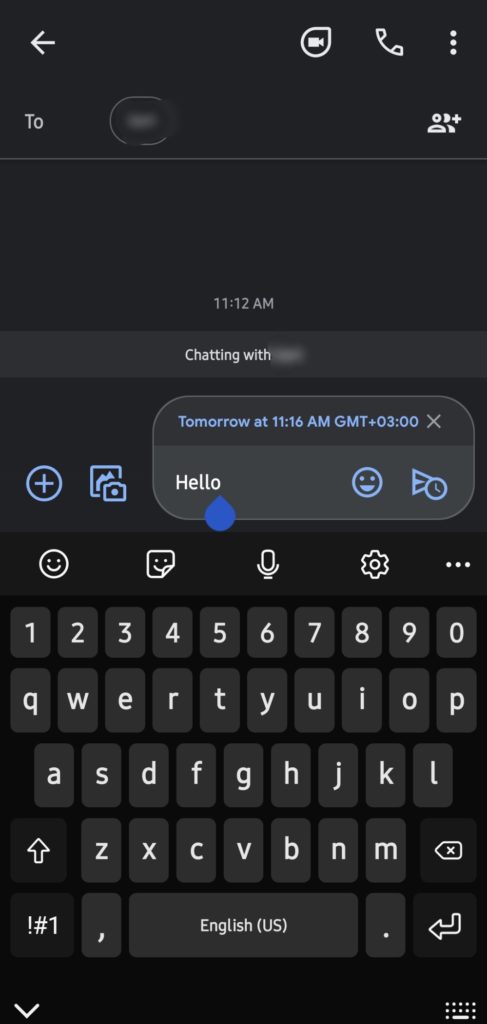In the image, a cell phone screen is displayed with an active chat interface. At the top of the screen, there is an arrow pointing to the left in the top-left corner. Next to it are a FaceTime icon, a call icon, and three vertical dots aligned horizontally. Below this, the line reads "Chatting with," followed by a blocked-out name.

To the right of the blocked-out name, there are a couple of profile icons. Below this line, the time "11:12 a.m." is shown. Underneath this, it again says "Chatting with," followed by the same blocked-out name, with an additional note saying "Tomorrow at 11:16 a.m. GMT+300" in blue text.

Further down, a message bubble displays the word "Hello," followed by a smiley face icon and a ribbon icon. To the left of this message, there is a light blue circle containing a plus sign. Below this, five icons are lined up horizontally: a gallery icon, an emoji icon, a gallery icon again, a microphone icon, and a settings icon followed by the three vertical dots.

At the bottom of the screen is a keyboard with gray buttons and white letters and numbers. The entire background of the image is black, providing contrast to the elements on the screen.